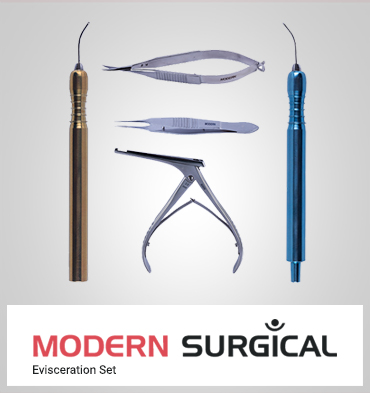The image depicts a collection of surgical tools arranged against a light gray background. On the far left, there is a gold-handled instrument with a thin metal pick extending from the top. To the far right, a similar instrument is present, but it features a metallic teal handle. Positioned between these two instruments are three silver tools. The topmost tool resembles a pair of pliers or grippers, characterized by two opposing curved bows that converge into a tweezer-like tip. The middle tool looks like a set of pointed tweezers. The bottom tool appears to have squeezable handles akin to a claw machine, suggesting a gripping function with a black slender rod or prong at the top. Below the image, a white band contains text: in large red capital letters, it reads "MODERN," followed by black capital letters spelling "SURGICAL." The dot of the 'I' in "SURGICAL" is stylized with a semicircular design underneath, resembling a person with outstretched arms. In the lower left corner, in small black text, it reads "evisceration set."